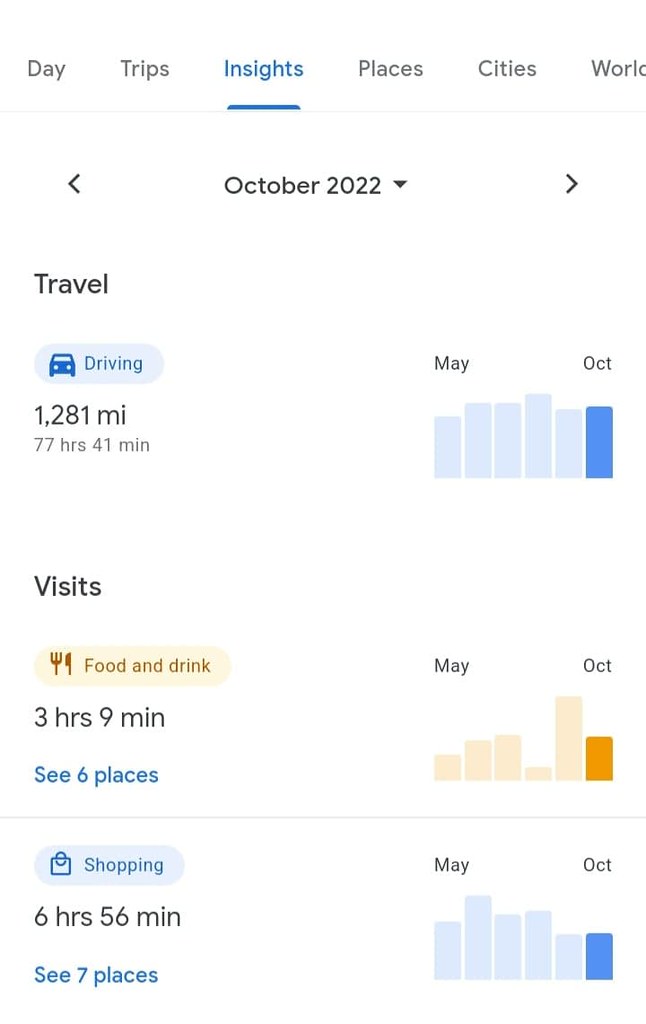This detailed itinerary displays an individual's travel activities for October 2022. The itinerary is formatted as a navigable menu, allowing users to explore day trips, insights, places, cities, and work. The travel category indicates that the person drove for a total of 77 hours and 41 minutes, covering a distance of 1,280 miles.

Their visits for the month totaled three hours and nine minutes, with an option to view the six specific places they visited. Additionally, there's a section for food and drinks, which can also be clicked on for more details. The shopping category reveals that they spent six hours and 56 minutes shopping throughout the month, with a clickable link to see seven different shopping locations.